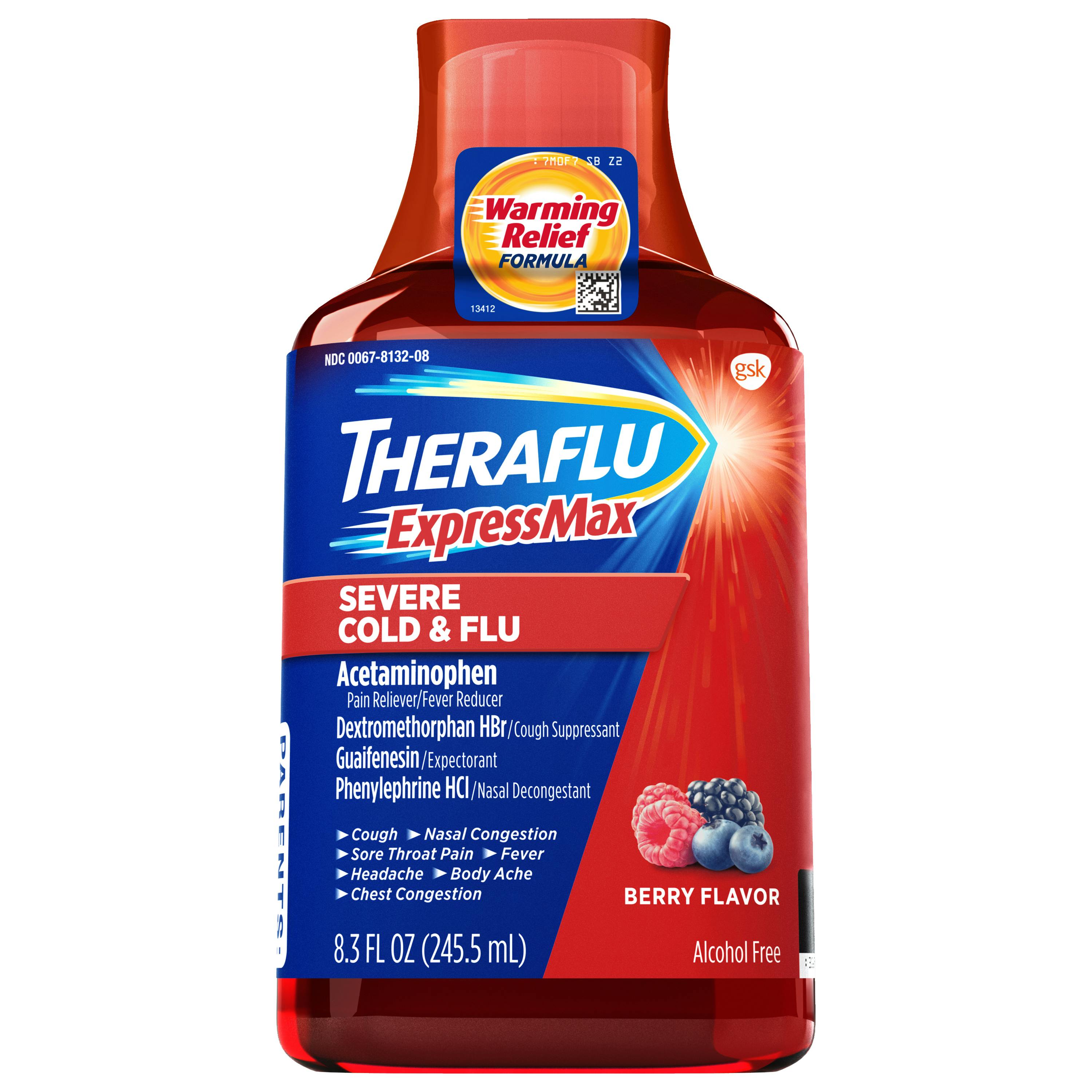This image depicts an 8.3-ounce bottle of TheraFlu ExpressMax, a severe cold and flu medicine. The bottle, which appears to be made of transparent plastic, contains red liquid and features a detailed label. Encompassing the bottle is a red wrapper with a prominent blue section at the top housing the product name "TheraFlu" in bold white text, and "Express Max" in red text. Below, "Severe Cold and Flu" is highlighted prominently, indicating its use for symptoms like cough, nasal congestion, sore throat, pain, fever, headache, body ache, and chest congestion. The lower section of the label specifies that the medicine is berry-flavored and alcohol-free, accompanied by images of various berries, such as raspberries, a blackberry, and blueberries. At the top of the bottle, a smaller label encircles the neck, stating "Warming Relief Formula" in red text with an orange outline. The red plastic lid, likely serving as a measuring cup, completes the packaging on this white background presentation.